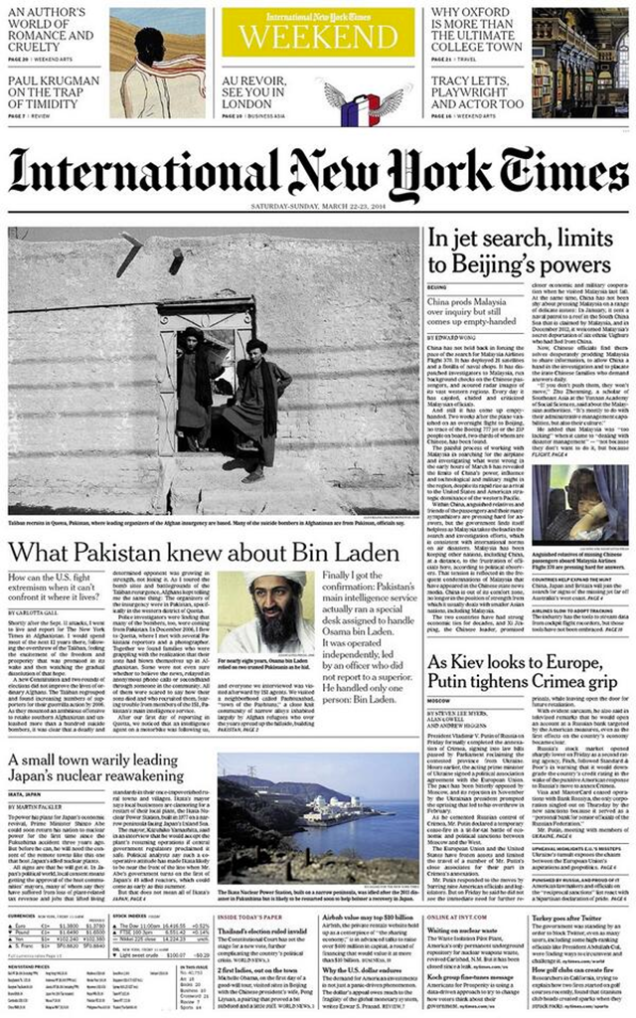This image depicts the cover of the International New York Times, dated Saturday to Sunday, March 22nd to 23rd, though the year is not clearly visible but appears to be a few years old. The newspaper header, "International New York Times," is prominently displayed at the top center against a yellow-orange background, beneath sections listing the content within the newspaper.

The front page features four primary articles. The main article, titled "What Pakistan Knew About Bin Laden," is the most prominent. Directly beneath this headline is an image of Osama bin Laden, while above it, another image shows the exterior of a building in Pakistan with two men in dark, traditional Pakistani attire standing in the doorway.

To the right of the lead article, another headline reads, "In Jet Search, Limits to Beijing's Powers," highlighting China's challenges in an ongoing investigation. Below this, another headline states, "As Kiev Looks to Europe, Putin Tightens Crimea Grip," focusing on geopolitical tensions involving Ukraine and Russia.

Lastly, positioned below the Bin Laden article, is another piece titled "A Small Town Wearily Leading Japan's Nuclear Re-," suggesting an ongoing narrative about a Japanese town coping with nuclear issues. The truncated headline implies the full text continues inside the newspaper.